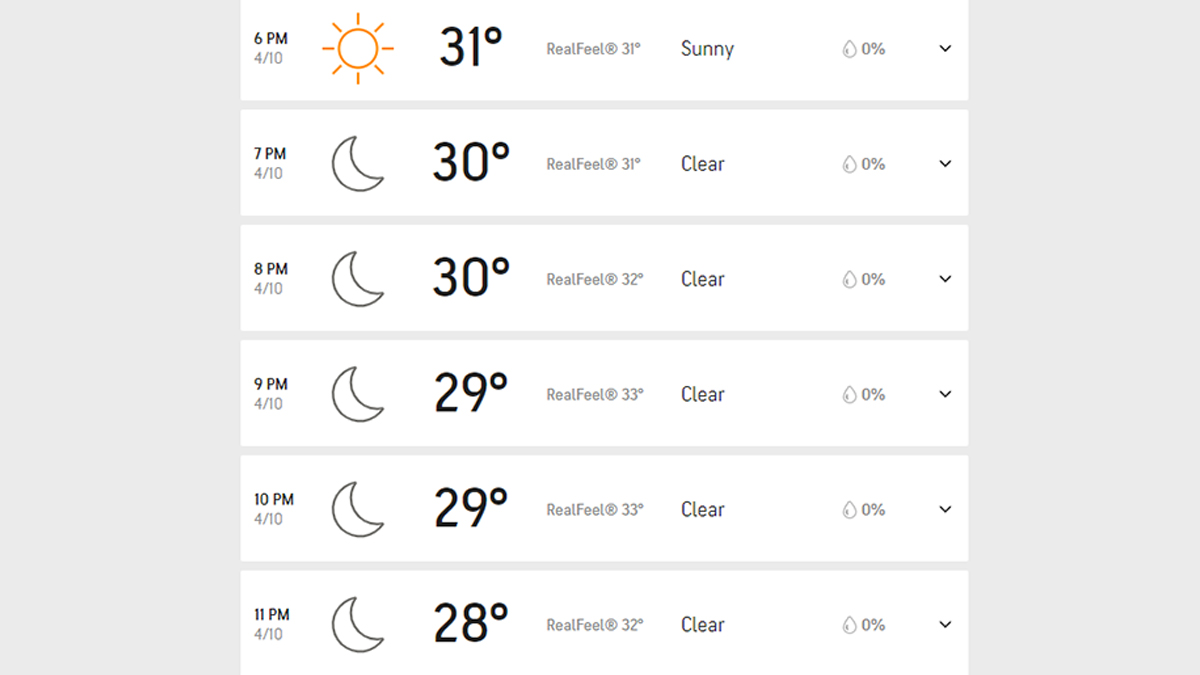This screenshot displays a detailed hourly temperature log for April 10th, spanning from 6 p.m. to 11 p.m. Each entry is organized into six distinct rows, with columns specifying the hour, an icon representing the time of day (sun or crescent moon), the recorded temperature, the "real feel" temperature, weather conditions, and precipitation levels.

- **6:00 p.m. (April 10th)**: Sunny, 31°F, feels like 31°F, sunny, 0% precipitation.
- **7:00 p.m. (April 10th)**: Clear with a crescent moon icon, 30°F, feels like 31°F, clear, 0% precipitation.
- **8:00 p.m. (April 10th)**: Clear with a crescent moon icon, 30°F, feels like 32°F, clear, 0% precipitation.
- **9:00 p.m. (April 10th)**: Clear with a crescent moon icon, 29°F, feels like 32°F, clear, 0% precipitation.
- **10:00 p.m. (April 10th)**: Clear with a crescent moon icon, 29°F, feels like 33°F, clear, 0% precipitation.
- **11:00 p.m. (April 10th)**: Clear with a crescent moon icon, 28°F, feels like 30°F, clear, 0% precipitation.

Each entry in the list is encapsulated in a clean, white box, ensuring clear visibility of the data. The temperature progression shows a slight decrease throughout the evening while maintaining consistent "clear" weather conditions with no precipitation.